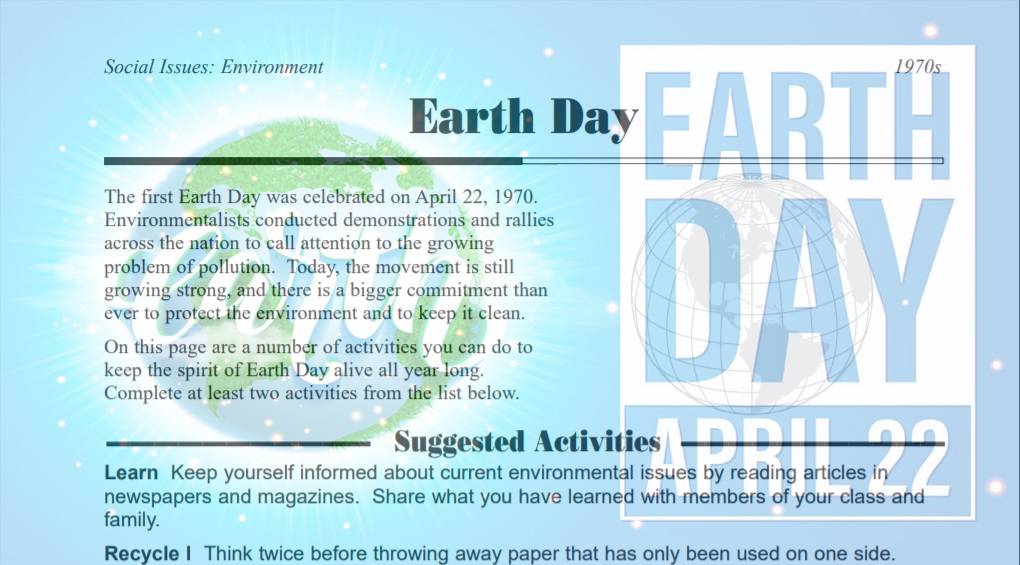**Earth Day Awareness Poster**

This Earth Day poster features a serene blue sky background and prominently displays an image of Earth. Overlaid on this image is the word "Earth" written in elegant cursive. Above the Earth, text highlights the historical significance of Earth Day, noting its inception on April 22nd, 1970, when environmentalists held demonstrations and rallies across the nation to bring attention to pollution issues. The text emphasizes the enduring strength and increasing commitment of the Earth Day movement, encouraging continual participation.

The poster lists several activities under a section titled "Keep the Spirit Alive." Suggested activities include staying informed about current environmental issues ("learn") and recycling. On the right, there is a faded depiction of another Earth Day poster from the 1970s, indicating what some of the original posters looked like during the early years of the movement. The overall design is accentuated by subtle rays of light emanating from the image of Earth, giving a radiant and hopeful aesthetic.

This poster serves as a powerful reminder of the ongoing efforts and dedication required to protect our planet, encouraging viewers to participate in Earth Day activities and educate themselves on environmental matters.